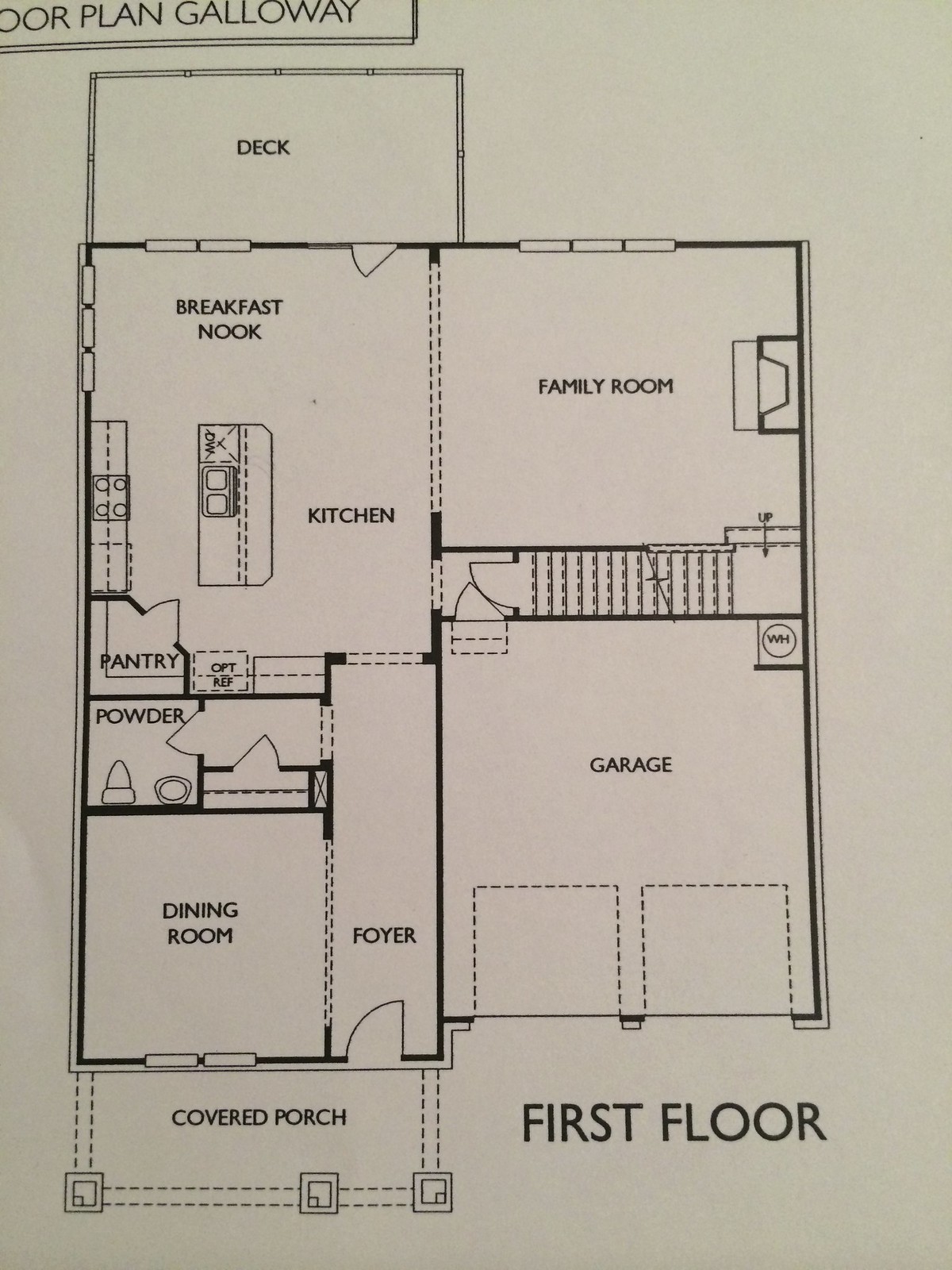This detailed floor plan illustrates the first floor of the Galloway home, meticulously drawn in black ink on white or beige paper. Although the title at the top is partially cut off, it is still identifiable as "Floor Plan Galloway." The layout forms a square area, with each space thoughtfully arranged for practicality and comfort.

Starting in the top left corner, the kitchen area features a charming breakfast nook and a convenient pantry. Directly to the right of the kitchen is a spacious family room, creating an open and welcoming area for family gatherings and relaxation.

A set of stairs is positioned adjacent to the family room, leading to the upper floors. Below the family room, there lies a two-car garage, complete with a door that provides access to the stairway landing, ensuring seamless entry into the kitchen.

To the bottom left, one can find the powder room, which is nestled between the dining room and the foyer. The dining room, situated next to the foyer, extends outdoors to a covered porch, offering an ideal space for alfresco dining or relaxation. Similarly, the breakfast nook of the kitchen opens up to a deck, perfect for enjoying a morning coffee or outdoor meals.

The kitchen is intelligently designed to share a wall with both the family room and the foyer, ensuring that all key living areas are easily accessible. Meanwhile, the foyer connects directly to the dining room, which, in turn, shares a wall with both the powder room and the kitchen.

This floor plan exemplifies a thoughtful and cohesive design, maximizing both functionality and comfort on the first floor of the Galloway home.